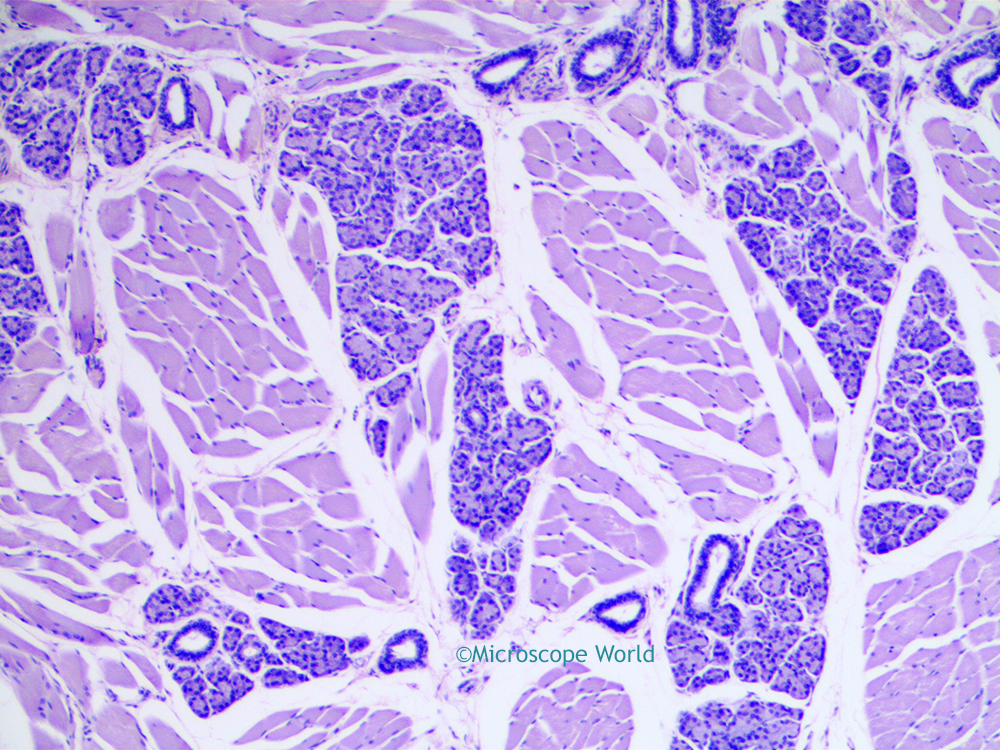The image is a large square microscope image with no border or text, featuring an abstract view of what appear to be cells. The background is primarily light purple, interspersed with darker purple patches. These purple sections, both light and dark, are irregularly shaped and outlined by thick white lines, resembling the marbled texture of a steak. Within these larger sections, there are thinner white lines creating intricate, seemingly random patterns. At the bottom of the image, printed in small green text, a copyright symbol is visible alongside the words "Microscope World," suggesting the source of the microscopic view.